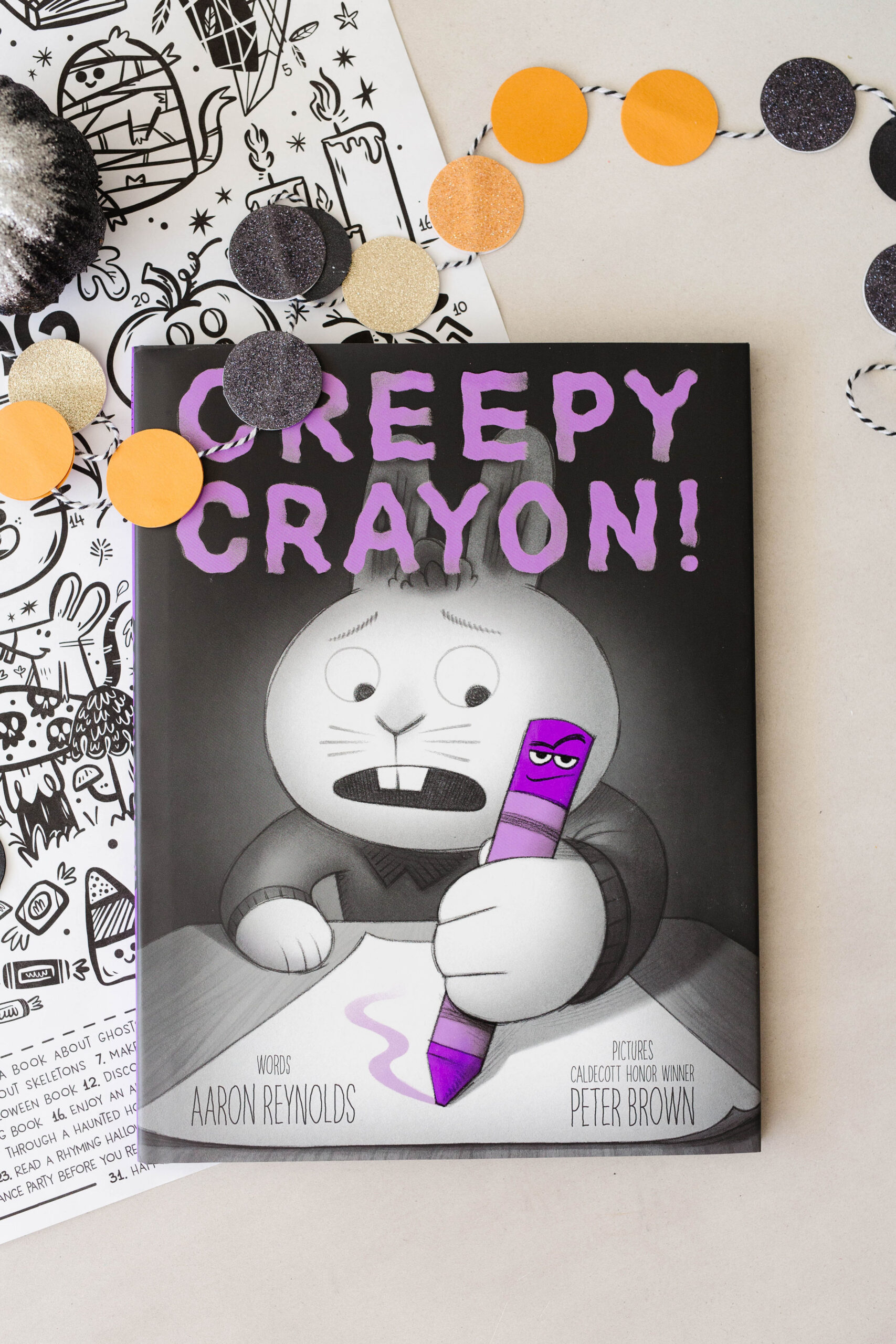The image is a detailed photograph of a book cover titled "Creepy Crayon!" drawn on a slightly reddish-gray paper, resting on a gray table. The center of the cover showcases a black-and-white, scared-looking rabbit with large, expressive eyes, furrowed brows, and an open mouth highlighting two trapezoid-shaped teeth. The rabbit, drawn in an oval-faced, cartoon style, has two vertical ears with a tuft of hair between them and is clad in a black jacket with one paw resting on the table.

The rabbit holds a purple crayon that bears a sarcastic expression with white eyes and a smirk. The crayon draws a squiggly purple line on a piece of what is presumably white paper but appears slightly gray in the photo. Above the illustration, the title "Creepy Crayon!" is prominently displayed in purple text, followed by the words "Words by Aaron Reynolds" on the right and "Pictures by Caldecott Honor winner Peter Brown" on the left.

Adjacent to the main illustration, there is an additional page featuring black-and-white Halloween-themed illustrations, including a candy corn, a mouse next to a mushroom, a candy, a pumpkin, and various obscured objects. An orange and black string garland decorates the background, looping around with alternating colored circles. The overall scene points towards a Halloween theme, creating a sense that the cover is aimed at children and possibly for a coloring book.